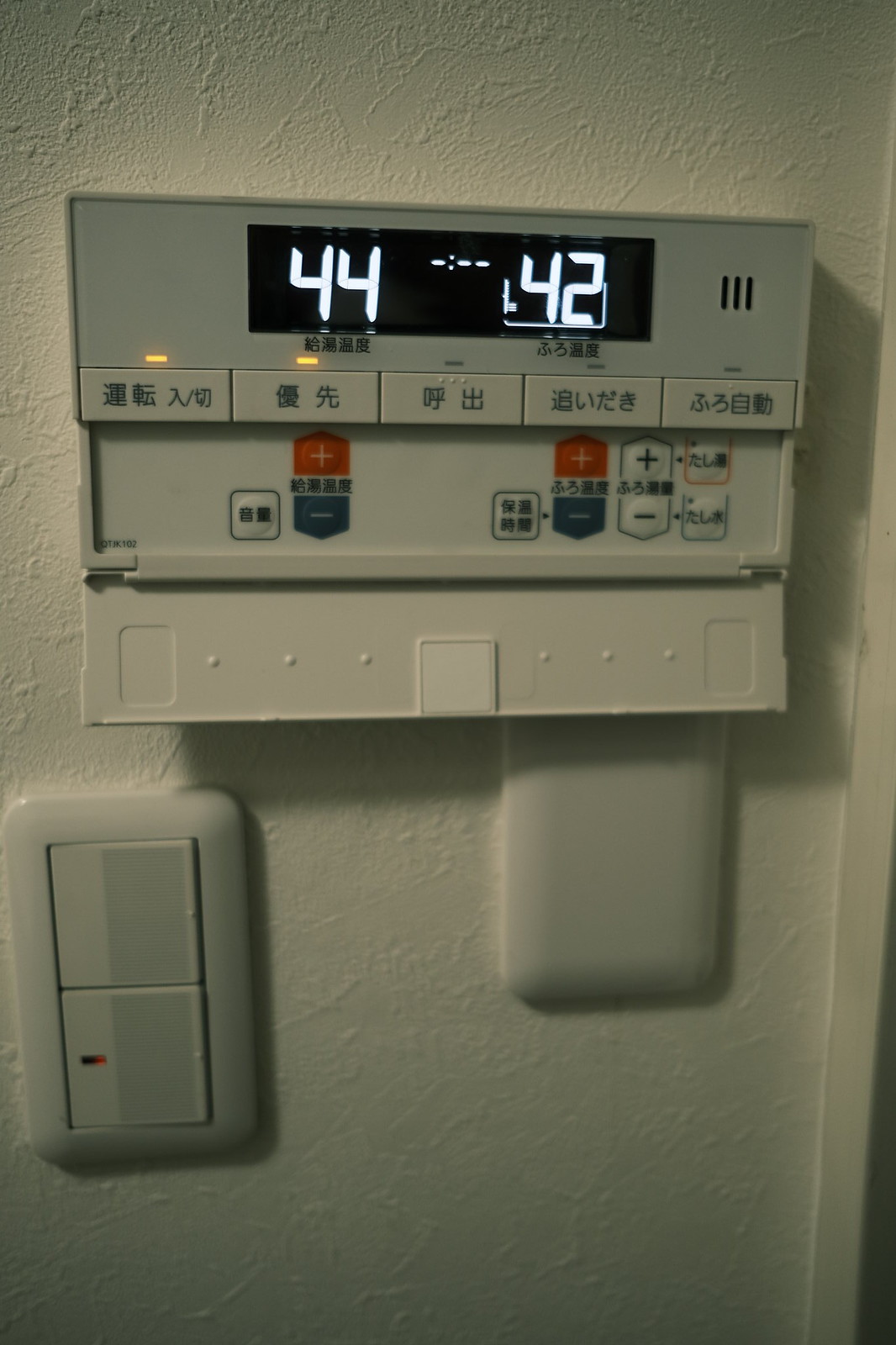The image depicts a white stucco wall featuring three distinct panels. 

In the bottom left section, there is a small panel with two unmarked buttons. The top button has a gray square on the right side, with what appears to be Braille indentations. The bottom button is nearly identical but has a sticker resembling an American flag. The panel lacks labels indicating the buttons' functions.

Towards the middle right of the image, there is another panel that appears blank, as if it has been either covered or conceals something.

The most detailed panel is situated at the top. This panel resembles an opened thermostat, revealing a digital display and multiple buttons. The digital display shows the numbers "44" on the left and "42" on the right. Centrally, the display features a spot that could be indicating the time or a countdown.

The middle section of this top panel contains five buttons, each with an indicator light. The two buttons on the left are illuminated, while the other three are not. Both the digital display and the buttons are marked with different Japanese characters. Below the opened panel, a button with more Japanese characters is visible, marked with a red plus sign and a blue minus sign. To the right of this button, there is a repeat of the plus and minus signs, but this time in white. Additionally, there is a white button outlined in red and another button outlined in blue.

Given the numbers "44" and "42" are displayed, and assuming these aren't temperature readings in Fahrenheit—since that would imply an excessively high temperature—the values might instead represent humidity levels.